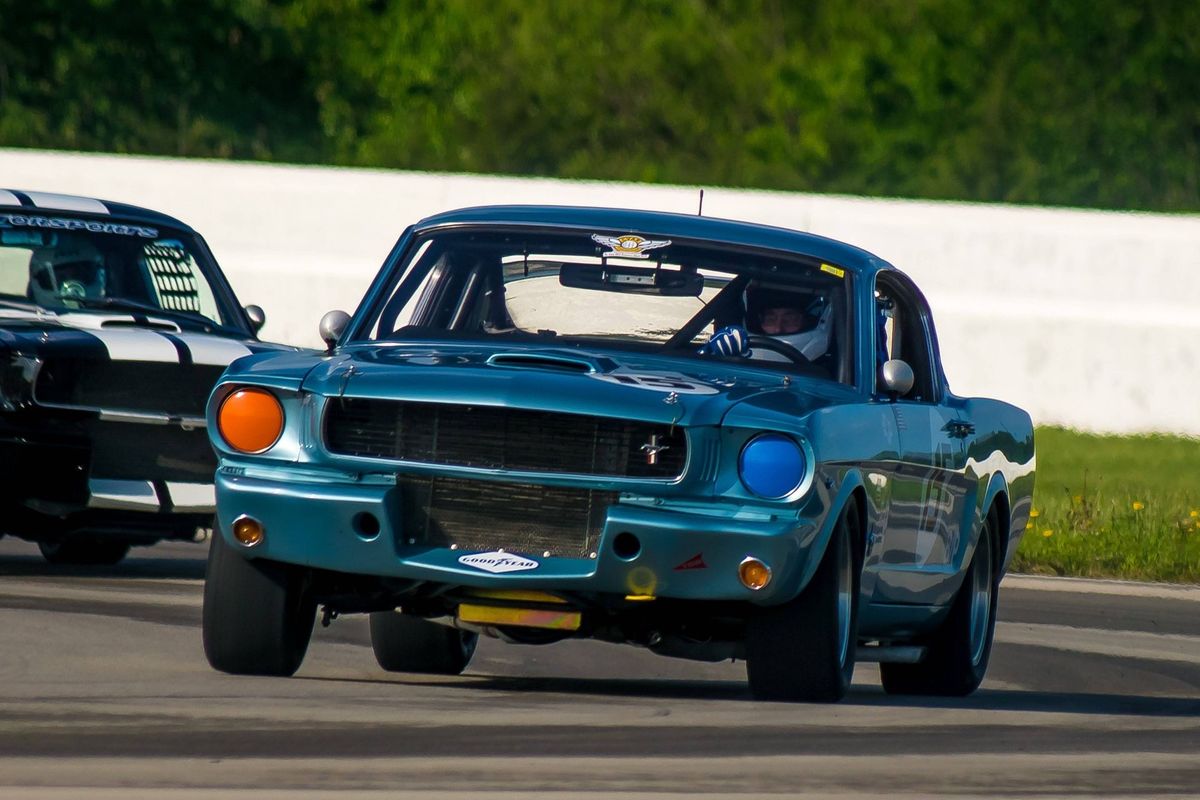The image showcases an intense racing scene featuring a heavily modified, dark blue Mustang, likely a GT350. The car has distinctive details such as mismatched headlights—blue on the right and orange on the left—and a cyan hood adorned with the number 15. The driver, visible through the windshield, is wearing a white helmet. A sticker reading "Goodyear" decorates the bottom grill of the Mustang. In the background, another car, identified as a black vehicle with twin white stripes, follows closely. The setting is a racetrack with a white barrier separating the track from a backdrop of blurred green trees and grass dotted with yellow wildflowers. The scene captures the dynamic essence of the race, highlighting the prominent colors of blue, black, white, green, and varying shades of gray.